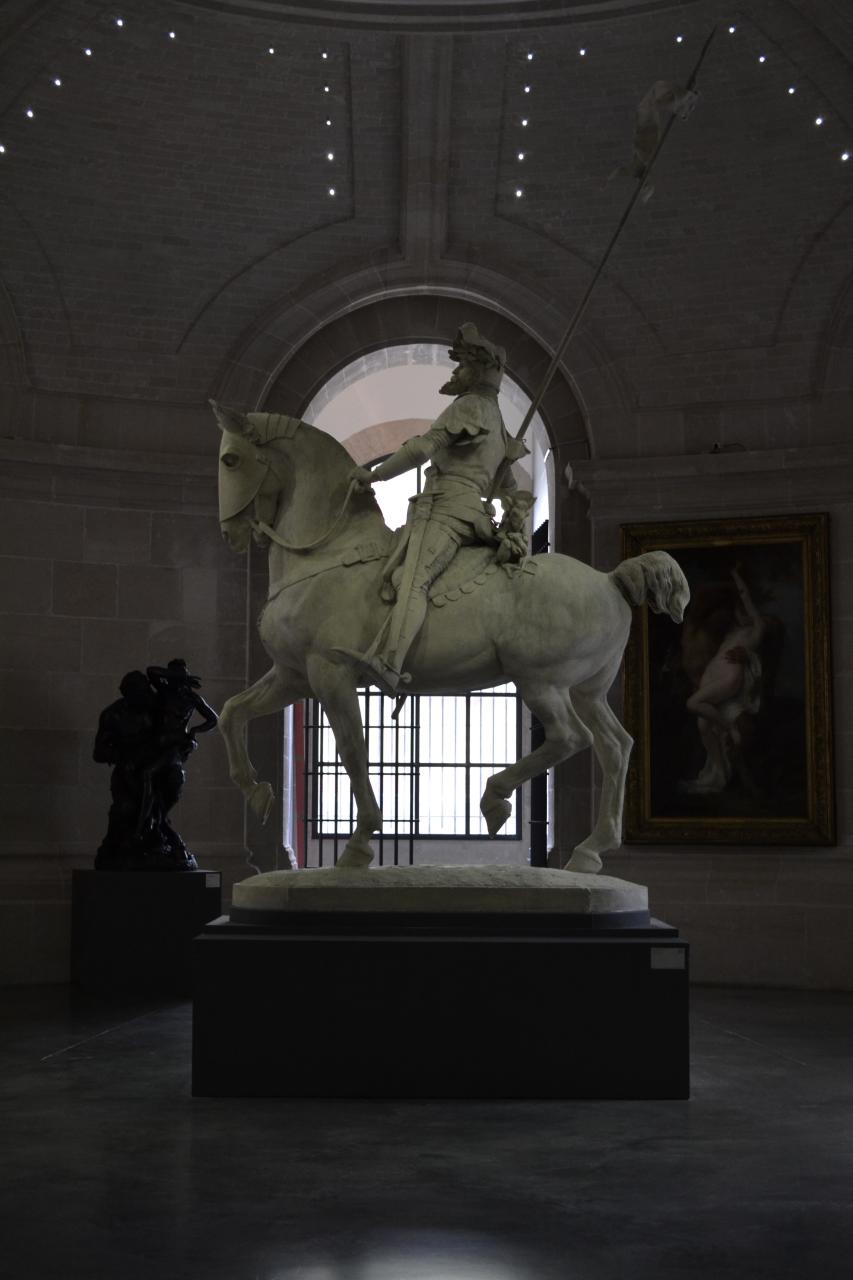The image shows an indoor photograph of a finely crafted statue, likely housed in a museum. The statue, displayed on a substantial black pedestal, depicts a soldier riding a horse, both rendered in striking white. The soldier is decked in war gear, including a helmet with a lifted visor, and appears to be holding the reins while sitting on a saddle. The horse is dynamically poised, with its front right leg and back left leg raised, conveying a sense of motion. Notably, the horse's face features a protective mask, and its tail is notably short. From a side profile view, the statue is illuminated modestly by a few ceiling lights and additional light filtering through an oval window and a barred window with some open sections. The ceiling above is intricate, featuring dotted lights in its cove. To the right, there is a barely-visible picture or drawing on the darkened wall, and to the left, a black statue structure provides additional context to the setting. There are no other people present in the image.